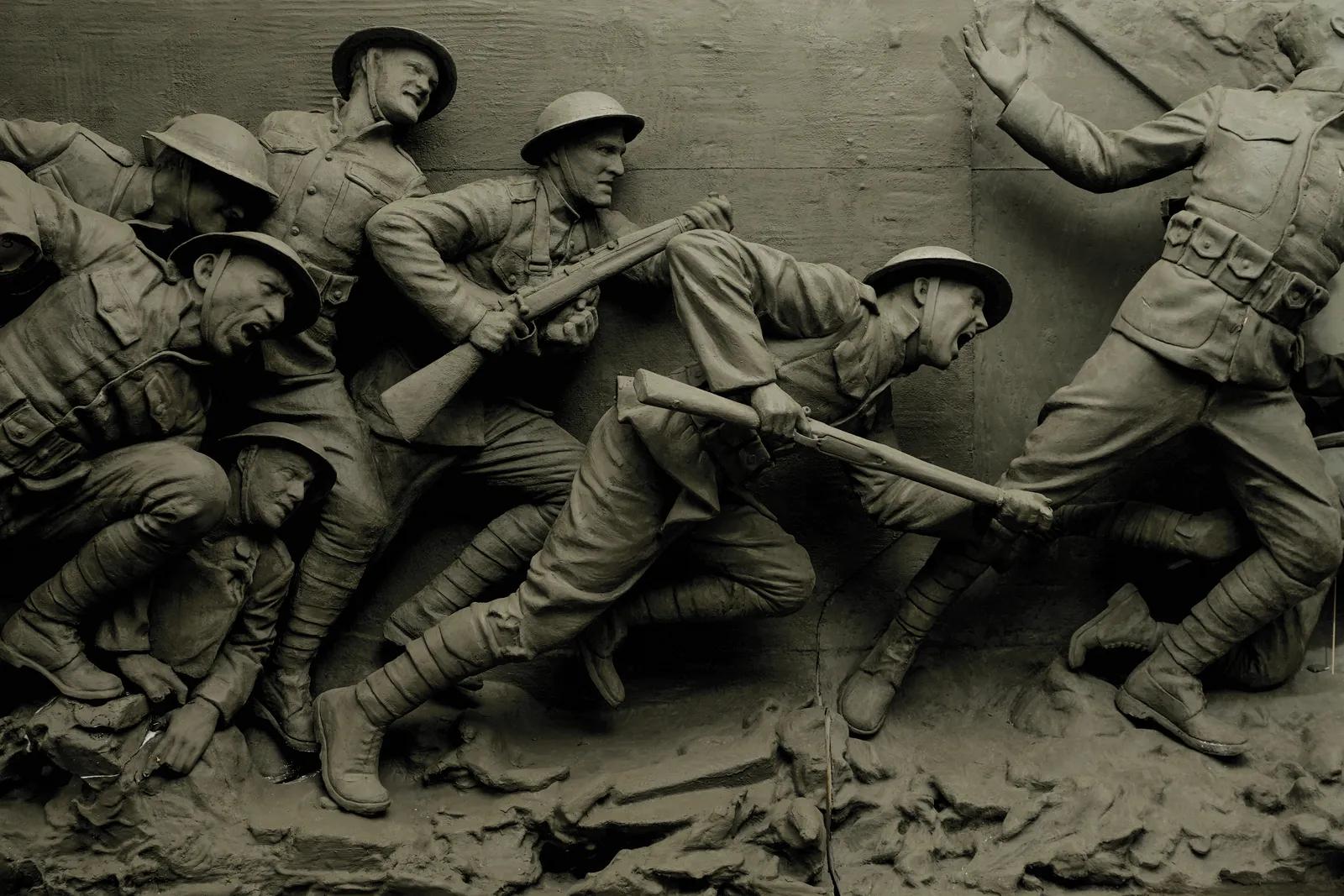This sculpture is an incredibly lifelike and detailed depiction of World War I soldiers, captured in a moment of intense action and emotion. The soldiers, approximately six visible, are engaged in a dynamic scene, moving from left to right. They are dressed in period-accurate Army fatigues, complete with long-sleeved jackets, pants, hard helmets with straps under their chins, and boots. Some soldiers also sport ammo belts and leggings. The central soldier appears to be lunging forward, gripping a rifle in his hands, his face intense with effort, almost as if screaming. The soldiers around him also carry M1 Garand single bolt-action rifles. The figure to the right has been injured, throwing his arms up and leaning back as if about to fall. 

The ground beneath them resembles a muddy, rocky terrain, suggestive of a battlefield strewn with obstacles. Behind them, a textured wooden trench wall, possibly sculpted with clay tools, adds depth to the scene, conveying the harsh, cramped conditions of trench warfare. The entire sculpture is rendered in a uniform brownish-gray color, which further enhances the realistic texture of the soldiers' uniforms and the surrounding environment, creating an overall impression that is strikingly lifelike and evocative of the grim realities of war.